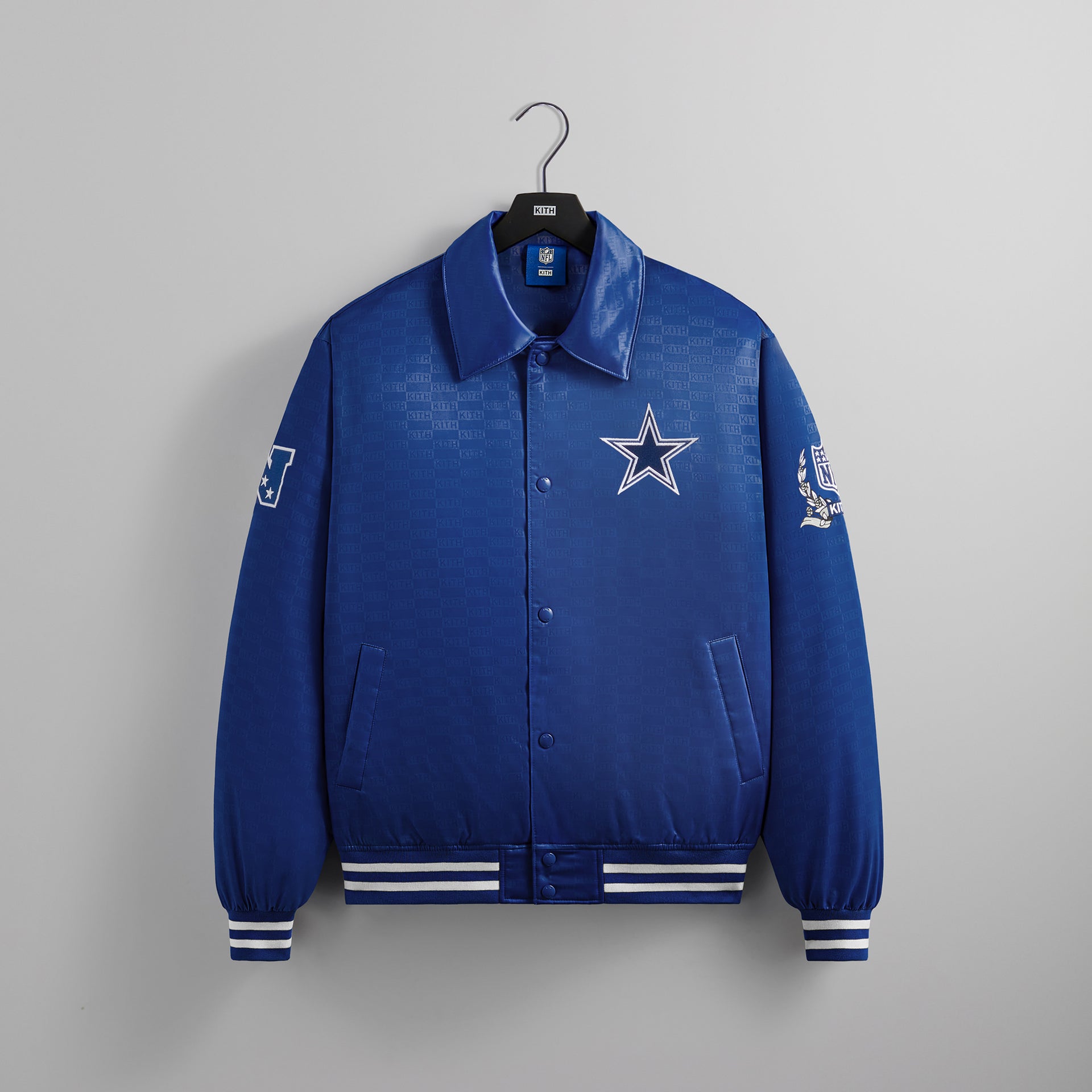The image features a distinct leather-like blue jacket, prominently displayed on a black hanger with a bent metal hook attached to a plastic section. The hanger curves to the left and is not suspended from anything, seemingly resting against a white background. A blue label reading "NFL" and a white rectangle with "K-I-T-H" in black text are visible on the back of the jacket. The jacket is adorned with an impressive repeating checkerboard pattern of the letters "K-I-T-H". It has six blue buttons along the front and a prominent blue star with a white border on the right breast pocket. The jacket also features two side pockets, white stripes around the hem and cuffs, and distinctive patches on the sleeves. The left sleeve boasts a star inside a shield, while the right sleeve displays a logo resembling the NFL emblem encircled by a wreath.